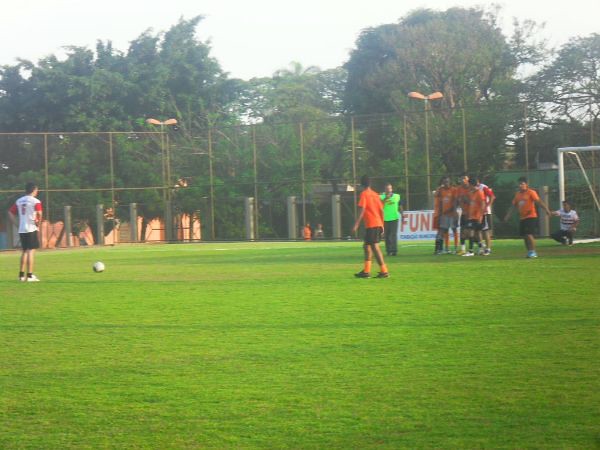The photograph captures a serene moment on a light green soccer field where players seem to be in a relaxed practice session rather than an intense match. Dominating the left side is a player donning a white and red jersey paired with black shorts, standing beside a white soccer ball. He is surrounded by teammates mostly clad in orange shirts and black shorts, who appear to be engaged in discussion. Not too far from them, a referee identifiable by his light green shirt and black pants observes the scene. To the right, a stark white goal post stands, near which a possible goalkeeper in a white t-shirt and black pants can be seen. Encasing the field is a tall, somewhat rusted chain-link fence, beyond which dense trees stretch across the background from left to right under a bright white sky. The image exudes the calm atmosphere of a typical training session under the open sky.